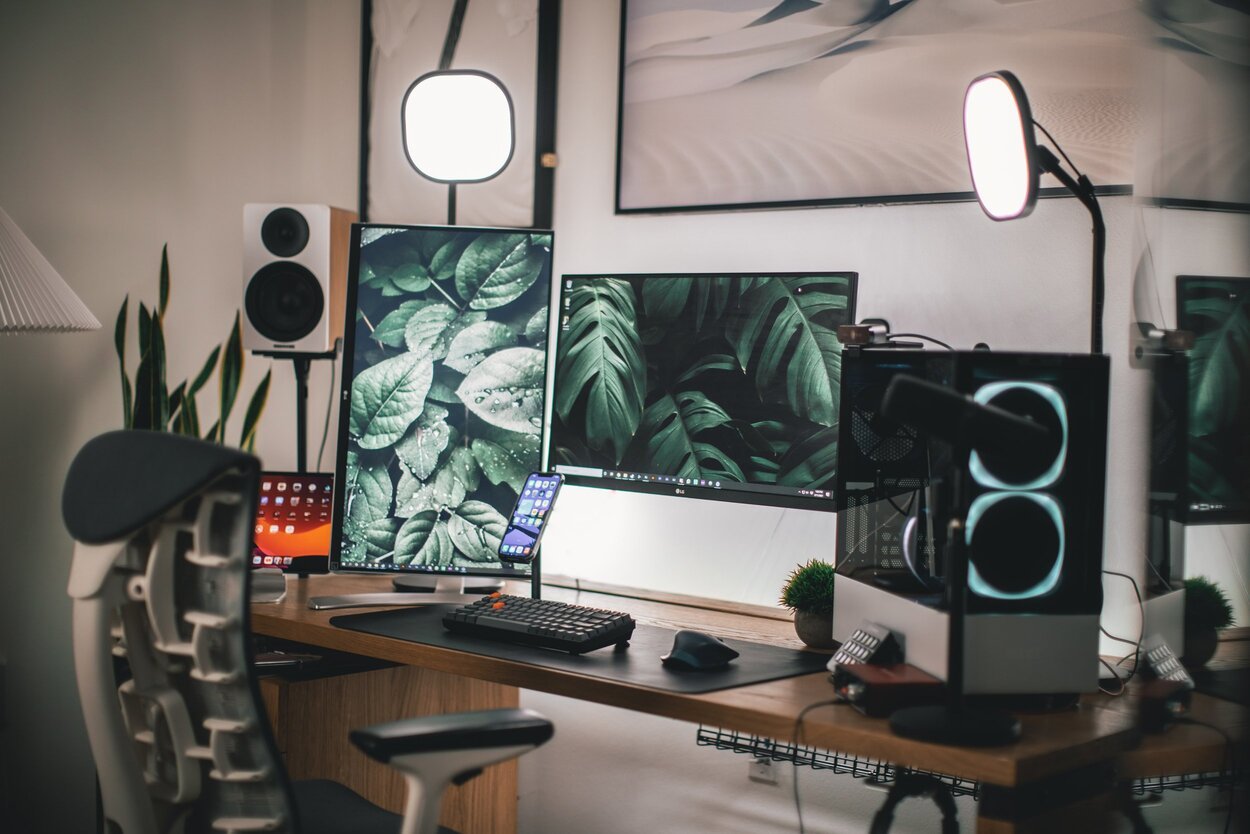The image showcases a sophisticated and modern computer setup in what appears to be a home office designed for video conferencing or filming. The setup features a minimalistic wooden desk pushed against a beige wall, adorned with a large, framed picture. On the desk, there are two large computer screens: one oriented vertically on the left and the other horizontally in the center. Additionally, there is a small tablet with a red screen on the far left side. Directly in front of the screens, a smartphone is placed on a stand, accompanied by a compact keyboard. To the right, a standard computer monitor and a computer base are situated. 

Prominently highlighted are two professional-grade, square lights on stalks behind the screens, purpose-built for optimal video lighting. A pair of large, black and white speakers are positioned on pedestals, complementing the black and white ergonomic chair that hints at extended use. A small, separate computer with a distinctive monitor displaying icons is also present. There is a plant peeking above the chair, adding a touch of nature to the technologically sophisticated workspace. This detailed arrangement clearly indicates a high-tech work environment tailored for extensive video conferencing or broadcasting activities.